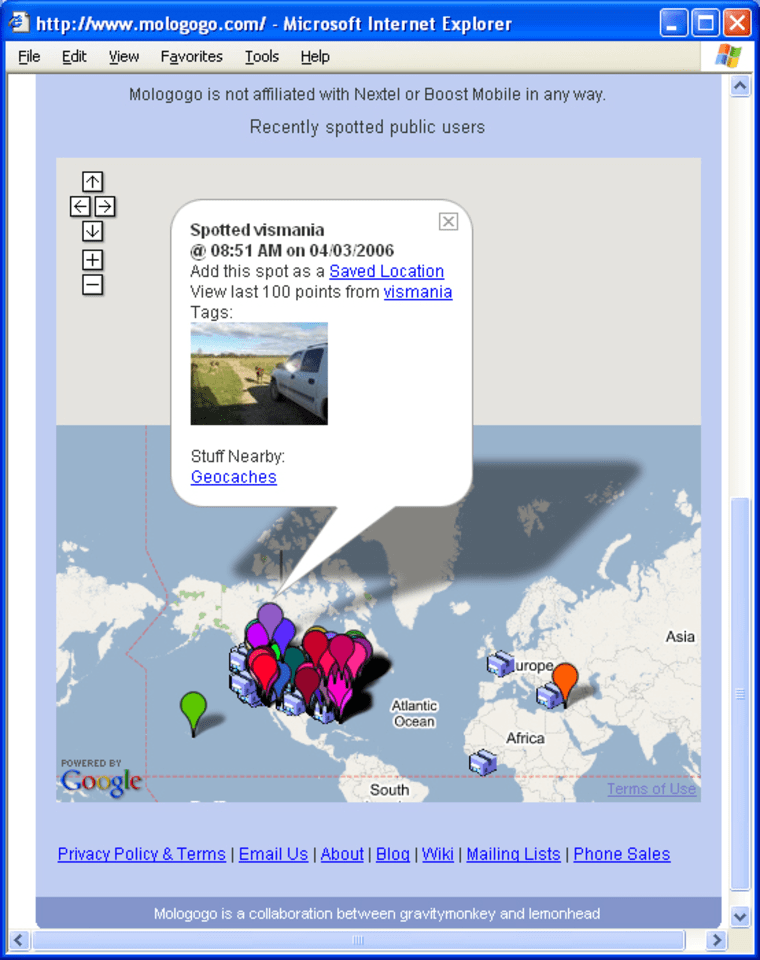The image appears to be a screenshot taken from a computer using Microsoft Internet Explorer, as indicated by the blue bar at the top displaying the URL "http://www.mologogo.com" along with the browser name. Below this bar, there's a gray menu section listing options such as File, Edit, View, Favorites, Tools, and Help.

Directly beneath this menu, a light blue section provides a disclaimer stating, "Mologogo is not affiliated with Nextel or Boost Mobile in any way," followed by a headline that reads, "Recently spotted public users."

The lower half of the image showcases a map of North America, densely dotted with various colored pin drops in purple, red, pink, and blue, indicating different locations. A rectangular pop-up is superimposed on the bottom part of the map, containing detailed information: it records a specific sighting timestamped at 8:51 AM on April 3, 2006, and offers options to "Add this spot as a saved location" or "View last 100 points from this mania tags."

To the side of this information box, there is a small image depicting a white car, seemingly driving on a road bordered by grass. Adjacent text mentions "stuff nearby geocaches," suggesting the presence of geocaching points of interest in the vicinity.